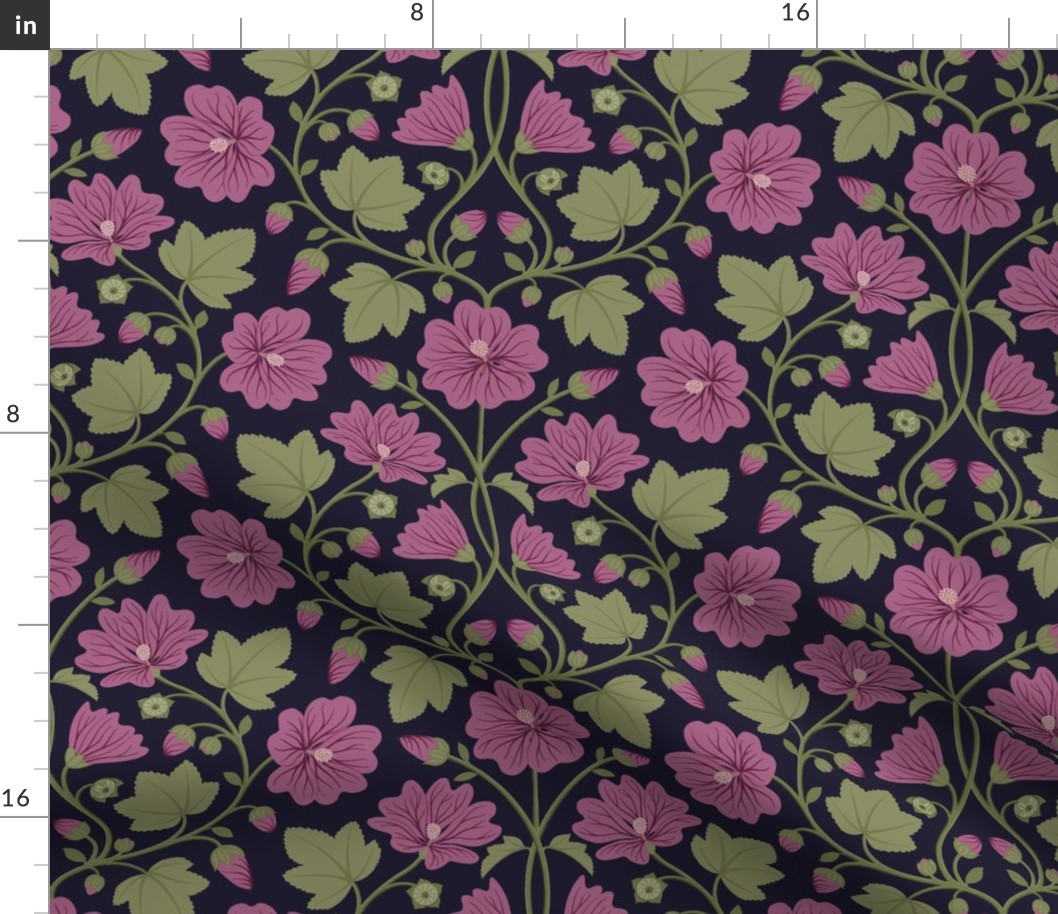This image features a dark navy blue fabric with an intricate and busy floral pattern. The background is either a very dark navy, dark purple, or black. Along the top and left-hand sides of the image, there are measurement markings with hash marks indicating inches. These measurements start in the upper left-hand corner, where a black square with white writing says "IN," likely indicating inches. Significant marks include the numbers 4, 8, and 16, with lines of varying lengths denoting each inch. The fabric appears to be approximately 17 or 18 inches square, perhaps slightly wider than it is long.

The floral pattern on the fabric is detailed and vibrant, featuring sage green to medium-light green leaves reminiscent of maple leaves intertwined like ivy. The flowers within the pattern are predominantly pink with some lavender or purplish hues. These flowers vary in stages of bloom, including both full blooms and buds with petals wrapped in a spiral ready to open. Elegant, curved stems connect the flowers and leaves, filling in most of the space and creating a densely packed design.